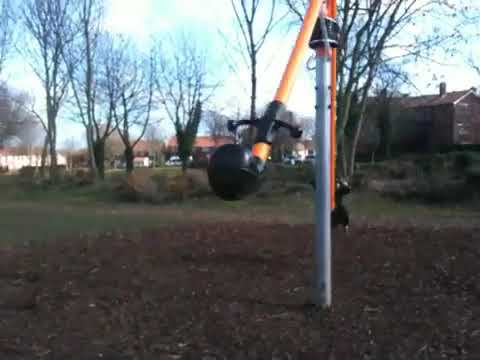The photograph captures an outdoor scene that appears to be set in a park or large backyard. The ground in the immediate foreground is covered in brown soil, transitioning to green grass further back. Positioned centrally on the brown soil is a tall white pole, likely cemented into the ground. Attached to the top of this white pole is an orange bar angled at approximately 90 degrees. At the end of the orange bar, there is a black, glove-like object. This structure could be an athletic or playground apparatus, suggesting it might be part of a larger recreational setup.

In the background, several dry, leafless trees rise behind the grassy area, possibly indicating the photo was taken in the fall or winter. Beyond the trees are a few houses; the one on the right is particularly notable, being a large brick house with a steep roof and chimney. The left side of the image contains more houses and some parked cars, adding to the residential feel of the setting. Overhead, the sky is a mixture of blue with scattered white clouds, emphasizing the outdoor ambiance.